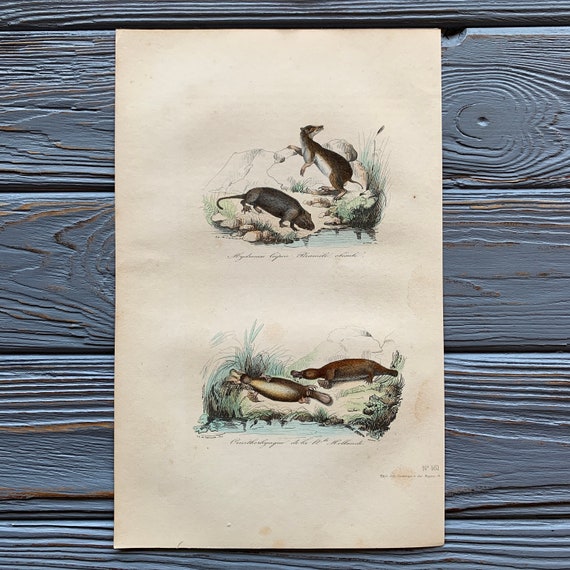This detailed color photograph showcases an old, slightly yellowed piece of paper, possibly stained from age or exposure to sunlight, lying on a wood-grain bench. The paper, displaying some warping, seems to have been partially in a frame or subjected to sunlight, as evident from the light and dark yellow markings along the right and bottom edges.

At the top of the paper, there are two finely drawn illustrations in pen and ink, featuring creatures that resemble black-furred rats or badgers. One is lying on its side, seemingly asleep on a rock, while the other, positioned to its upper right, appears to be lying down but with its head raised, gazing upward to the right. This scene is set amidst some rocks, greenery, and a hint of water, creating the impression of a natural habitat.

Below this, the second illustration presents a side view of what look like brown platypuses or similar sea creatures, both asleep on their sides, amidst tall grass with a rock in the background. There is a wash of color over portions of these detailed drawings, including blue water in the lower scene, and some hills suggested in the background. Italicized text, in light gray, is seen underneath each image, adding a touch of narrative to the composition.